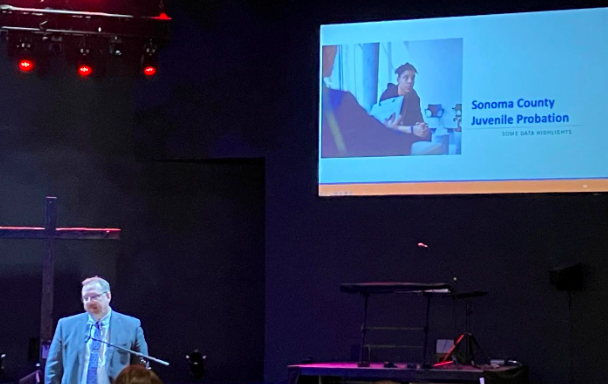The image captures a scene from an event where a middle-aged man is delivering a speech from a stage. Standing in the lower left corner, he is dressed in a gray suit with a white shirt and a blue tie, complemented by glasses and possibly a mustache. He is positioned behind a small podium with a long microphone, engaging with the audience. The backdrop features a wooden cross, suggesting this could be taking place in a church setting. Bright red lights from three track spotlights illuminate the stage, cutting through the otherwise dark, almost black, background. To the right, a large screen projects a white slide with the header "Sonoma County Juvenile Probation" and an image of a young individual. Additionally, a musical keyboard rests on a platform, further hinting at a multi-purpose venue. The detailed setup indicates the man may be presenting at a formal lecture or community meeting, potentially addressing issues related to juvenile probation.